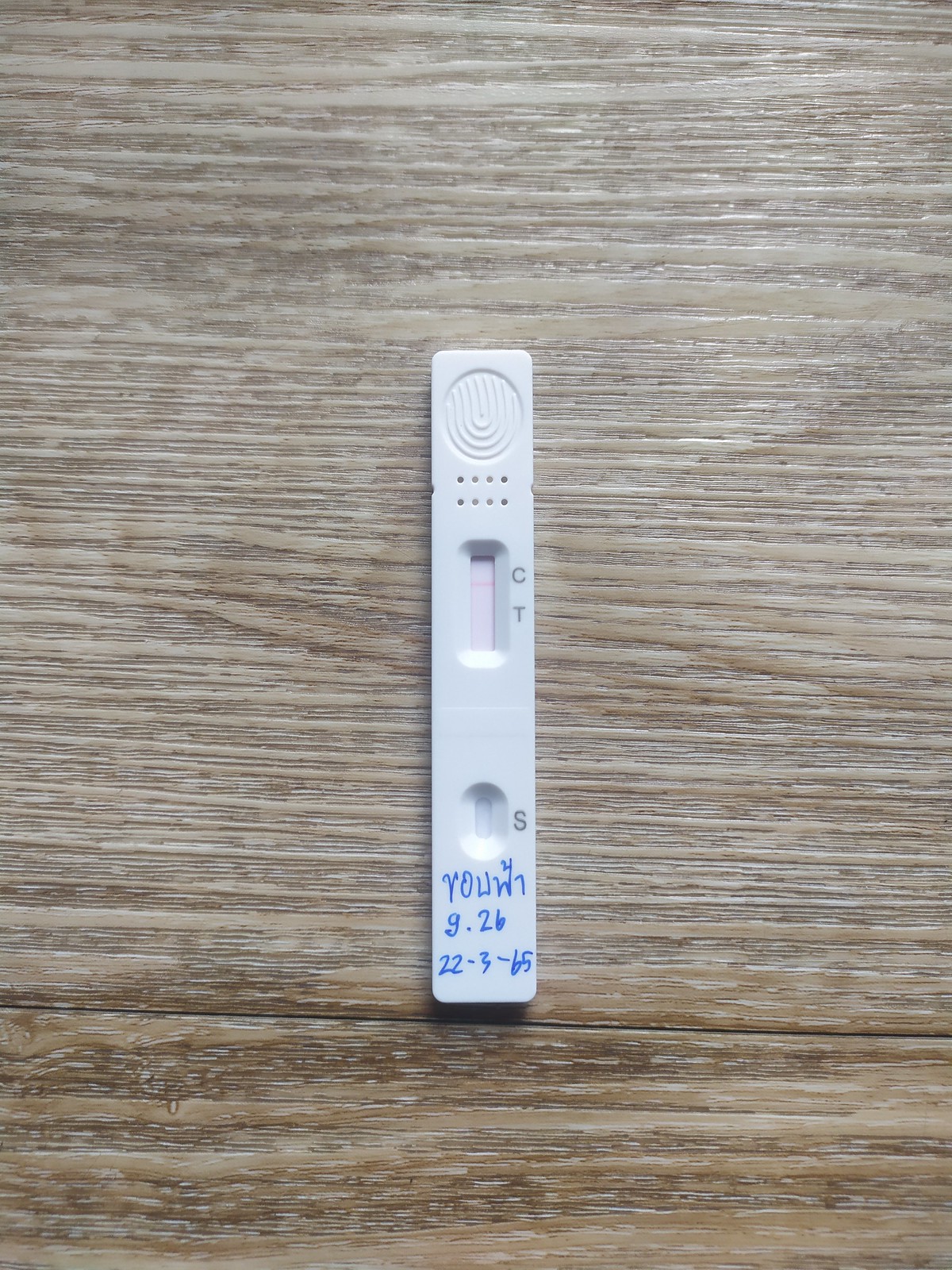This image features a small, rectangular white plastic device, likely a medical diagnostic test. Measuring approximately 2-3 inches in length, the top of the device includes an indented window displaying two faint red lines aligned with the letters "C" (control) and "T" (test). Further down, there is a circular hole labeled with the letter "S," which does not contain any colored marking. Below this, handwritten notations in blue ink can be observed, reading "YOU," a symbol resembling "W7," "9.26," and a date marked as "22-3-65" (March 22, 1965). The top of the device features a thumbprint-like design and is punctuated by two parallel lines of small holes. The device rests on a gray wooden table, adding contrast to its white color.